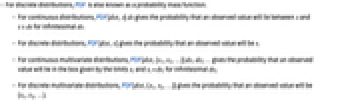This image is a partial screenshot of a document, showcasing a top section with text that is unfortunately too blurry to read, even when zoomed in. The text, predominantly in black with one blue word per sentence, is composed of one full sentence at the top, followed by four bullet-pointed sentences. These bullets are represented by dashed lines rather than traditional circles. The section of text takes up the top half of the image, set against a white background, with the bottom half of the screenshot being entirely blank. The font size is relatively small, and there are no graphics or other visual elements in the image.